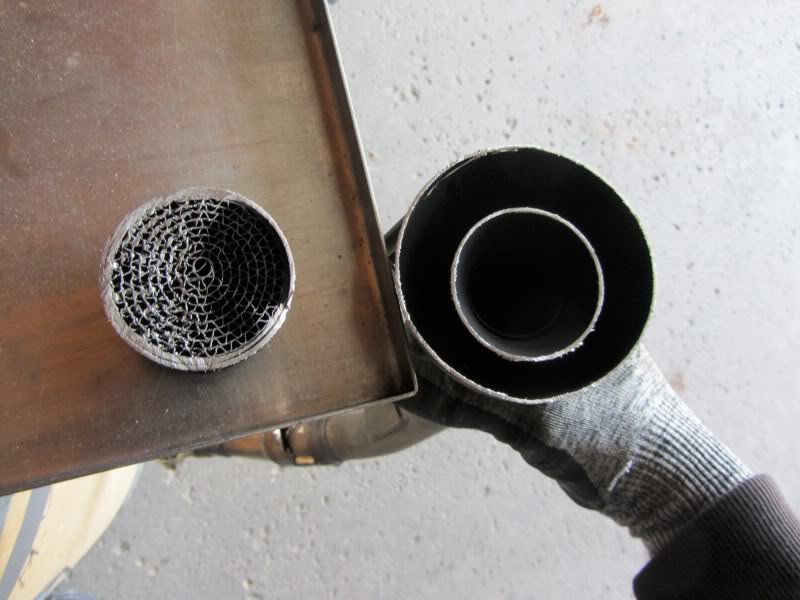The image depicts a room with a grey concrete floor featuring scattered spots. A person is visible, wearing a grey glove adorned with small rivets on its edge. The person's grey coat sleeve is visible, extending towards a greyish table. To the left side of the frame, a cone with webbing is present. On the right side, a greyish pipe is noticeable, within which a copper pipe runs vertically down, slightly below the table's surface.